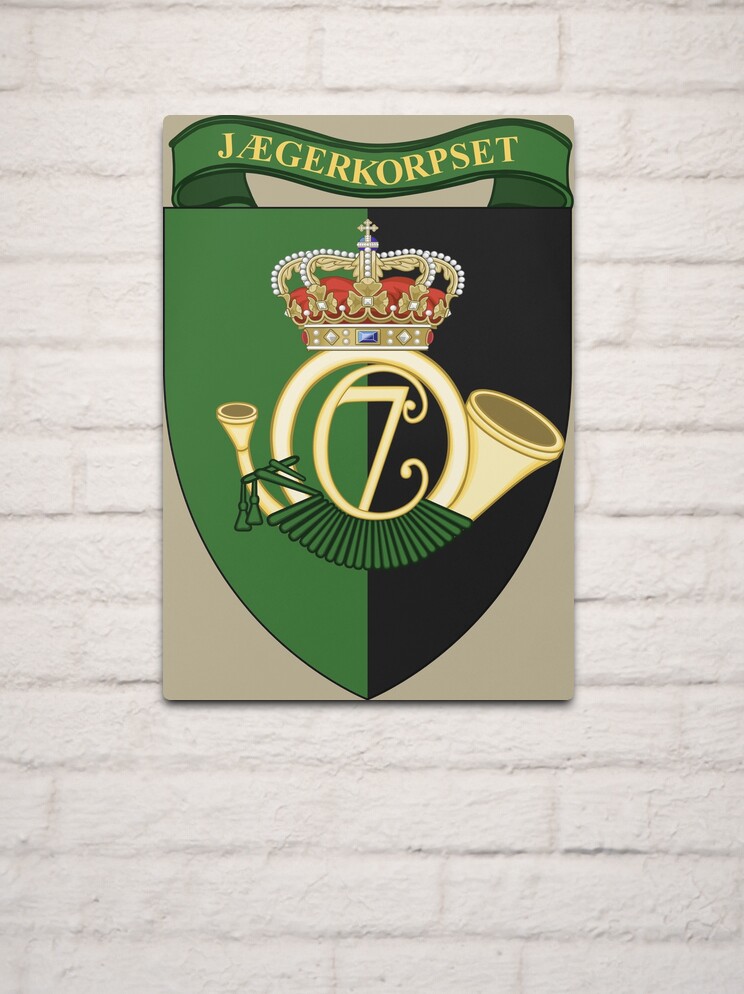The image showcases a white brick wall adorned with a plaque set against a gray background. Prominently featured on the plaque is a large green and black crest. At the top of the plaque, there's a green flag with yellow text that reads "Jaeger Korpsit." The crest itself is detailed and ornate, featuring a gold crown encrusted with various jewels, including a central red jewel, blue stones along the base, and smaller diamonds. Above the crown are two small crosses. Wrapped around the crest is a gold flugelhorn intertwined with green cord. At the center of the flugelhorn is a prominent gold "7."